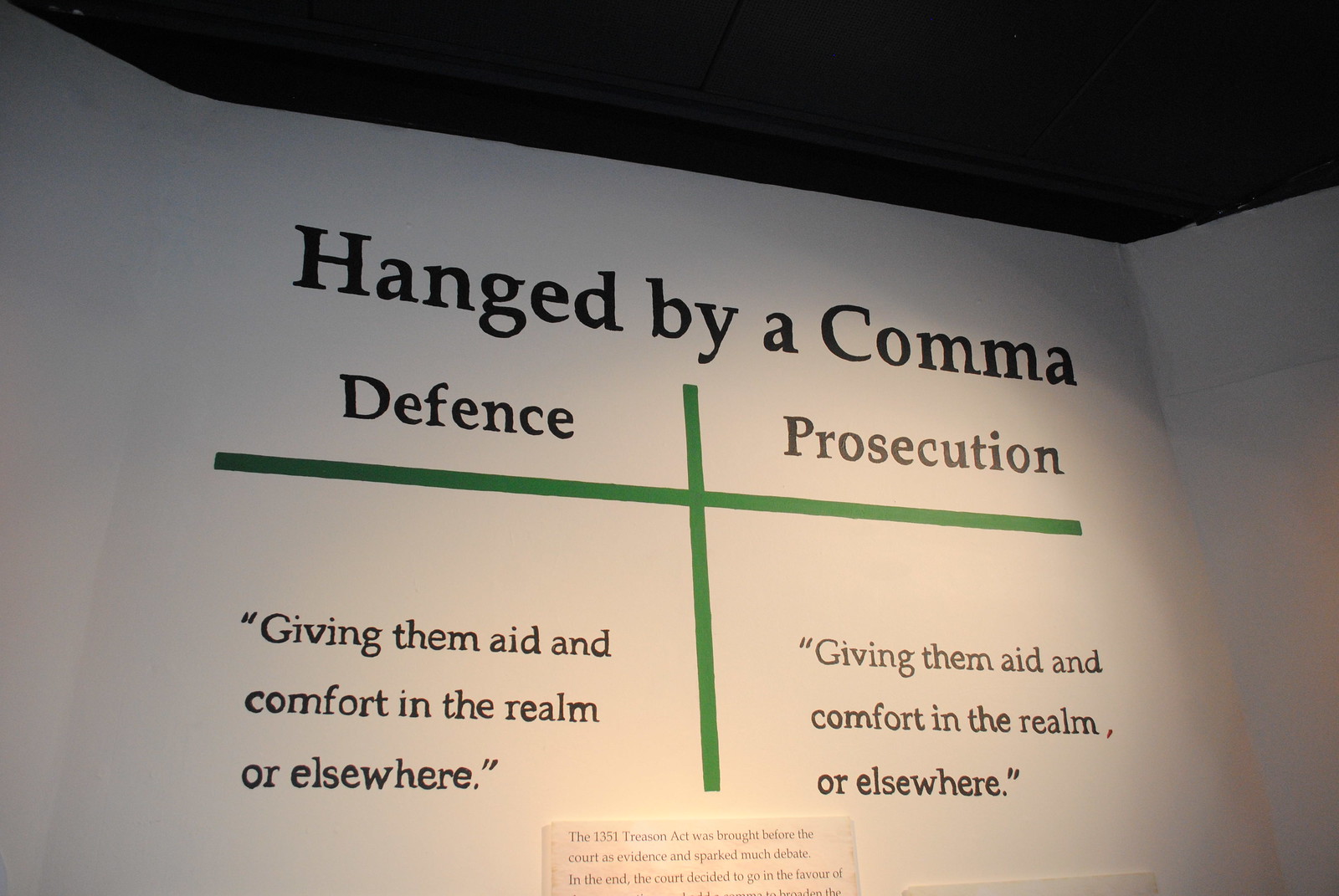On a white background resembling folded paper, the top black section bears the bold title, "Hanged by a comma." Below, a green cross-like figure with a short vertical and a long horizontal part divides the image into two columns. The left column is titled "Defense" and the right "Prosecution." Each column contains the identical phrase, "giving them aid and comfort in the realm or elsewhere," enclosed in quotation marks. At the bottom of the image, amidst a barely visible tag, a black or brown text on a tan background states, "The 1351 Treason Act was brought before the court as evidence and sparked much debate, in the end, the court decided to go in favor of..." before being cut off.